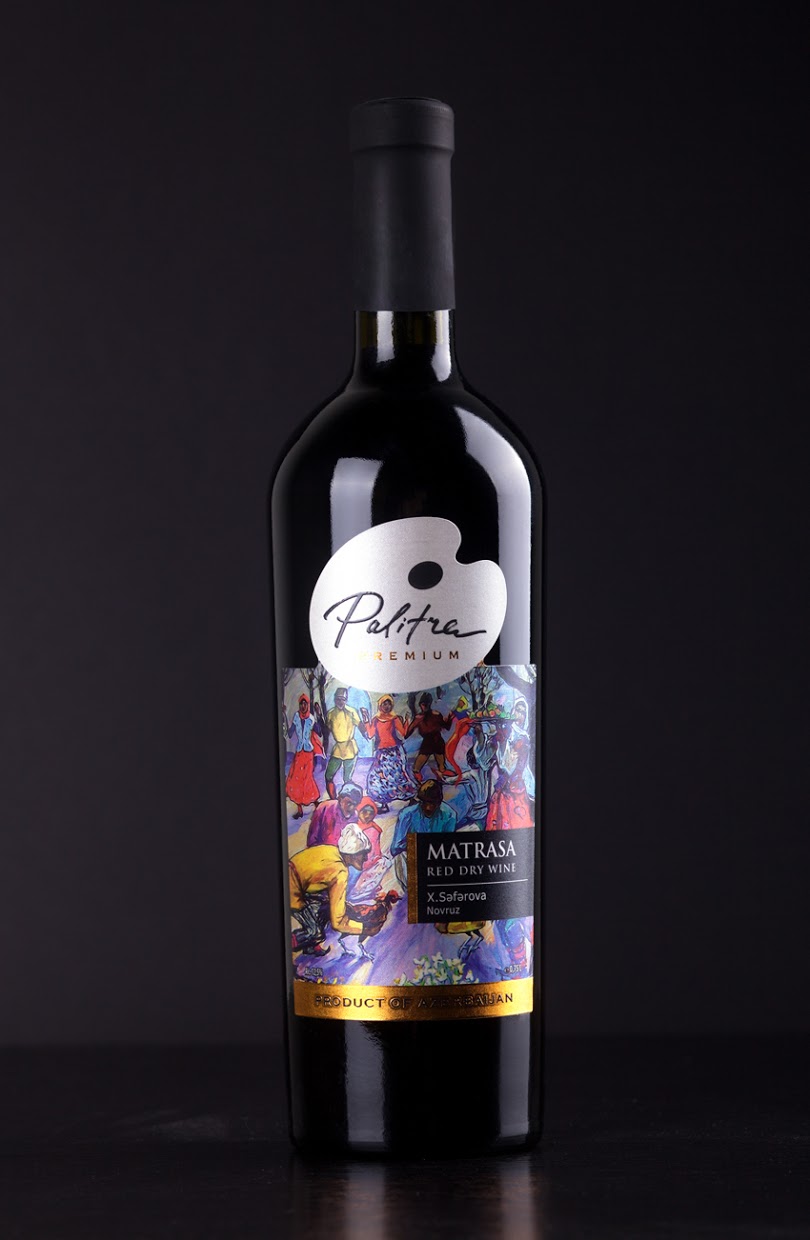The photograph features an elegant wine bottle from the Pelletreux Premium vineyard, characterized by its dark, sleek appearance against a somber black table and wall backdrop. The bottle's black glass exudes a reflective sheen, enhanced by its black foil-covered neck. Central to the wine bottle is a vibrant, dynamic label depicting a lively scene of black women adorned in an array of colorful clothing, including yellows, blues, and reds, some with floral prints. The women appear to be engaged in various activities, with a few dancing and one holding a chicken, and many wearing headscarves. Above this vivid artwork is a white painter's palette marked with the name "Pelletreux Premium," where 'Pelletreux' is inscribed in black and 'Premium' in gold text. The label also mentions "Matrasa Red Dry Wine," indicating the varietal, and a horizontal gold band at the bottom hints at the wine's origin, although the specific country is hard to discern. The striking contrast of the label's colorful imagery set against the bottle's dark background creates an eye-catching effect, making it an enticing showcase item, possibly intended to draw attention in a wine store setting.